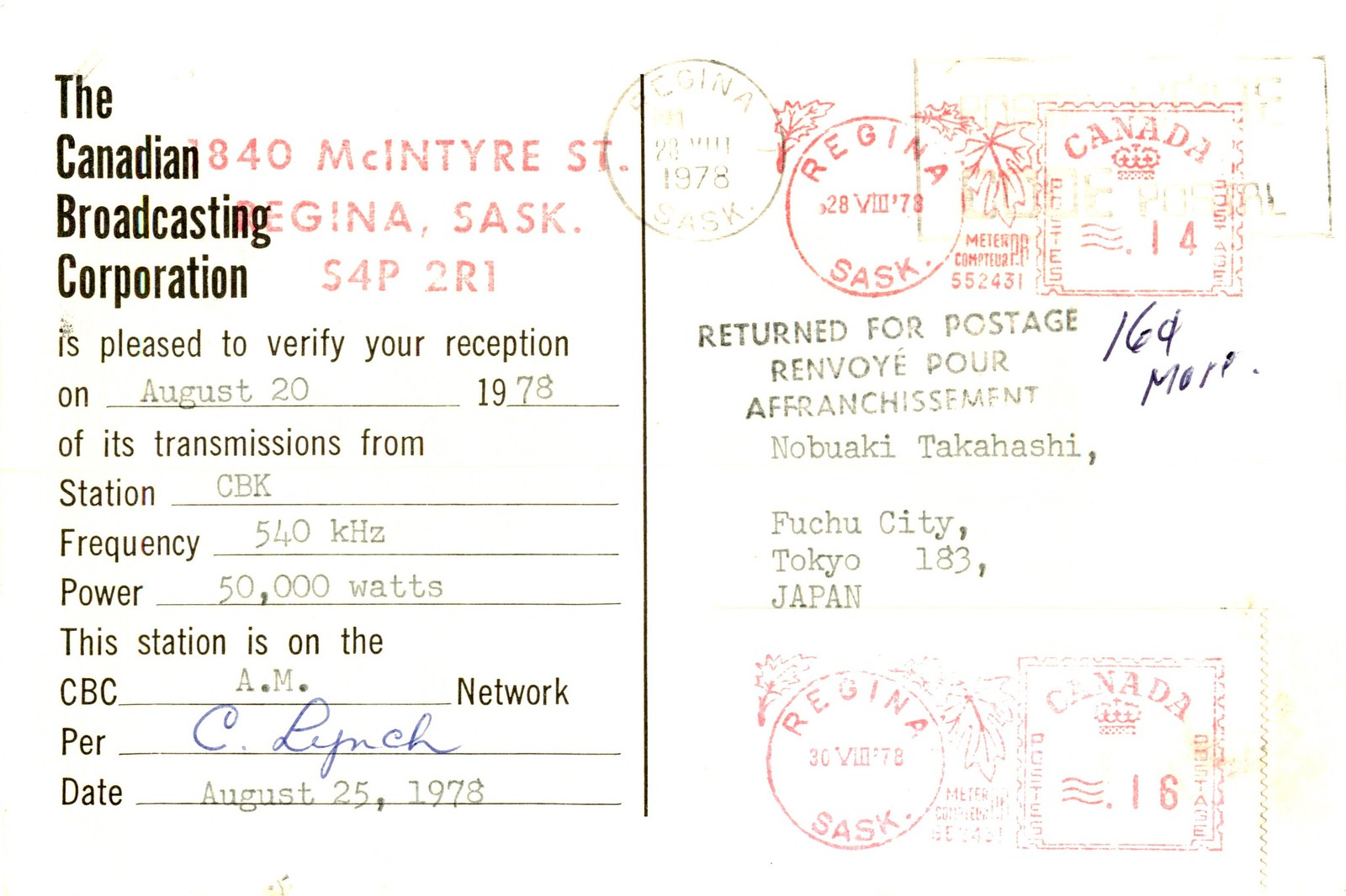A vintage postcard from the Canadian Broadcasting Corporation, dated August 25, 1978, showcasing a verification of reception for a broadcast on August 20, 1978. The postcard indicates the reception of transmissions from station CBK on a frequency of 540 kilohertz, with a power of 50,000 watts, which is part of the CBC AM network. The message is signed by C. Lynch. The right side of the postcard is adorned with multiple stamps, including several from Regina and a couple from Canada. Additionally, there is a "Return for Postage" stamp and some inscriptions in French. The postcard is addressed to Nobuaki Takahashi in Fuchu City, Tokyo 183, Japan.